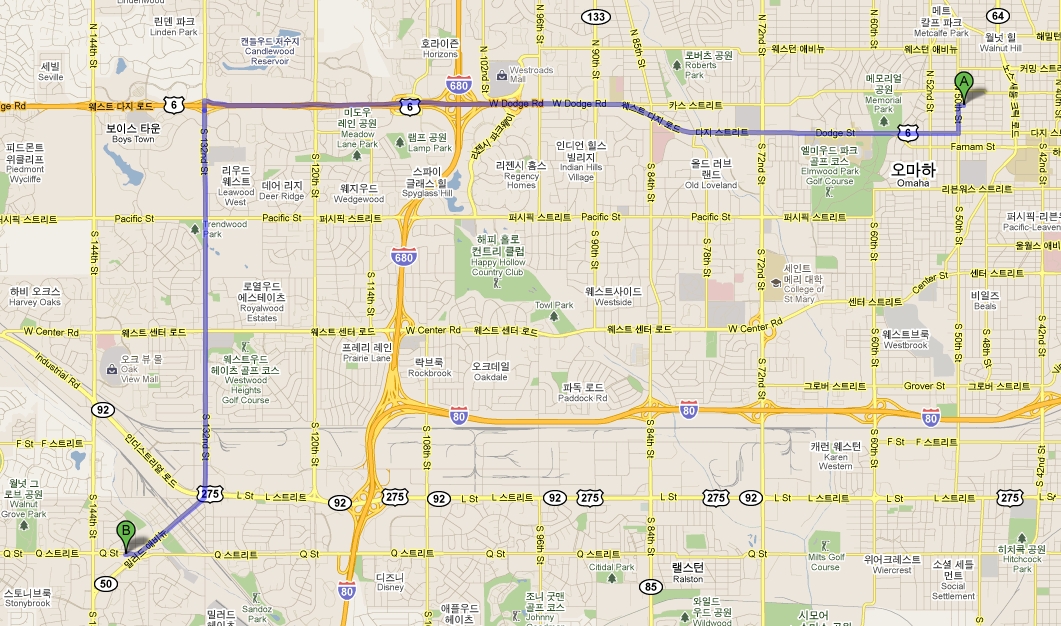A detailed screenshot of a map from Google Maps, displaying a section of Omaha, Nebraska, zoomed in closely. The map features bilingual labels, with place names and streets marked both in English and Korean Hangul. For example, the city name "Omaha" appears in English with larger Hangul characters above it. A routed path is mapped out, indicating directions from Point A to Point B. Point A is situated near the top right corner, close to the intersection of 50th Street and an unlabeled street, near Farnham Street. The path tracks west along Highway 6, then south along 132nd Street, finally reaching Point B at the bottom left corner, at the intersection of Q Street and South 144th Street.